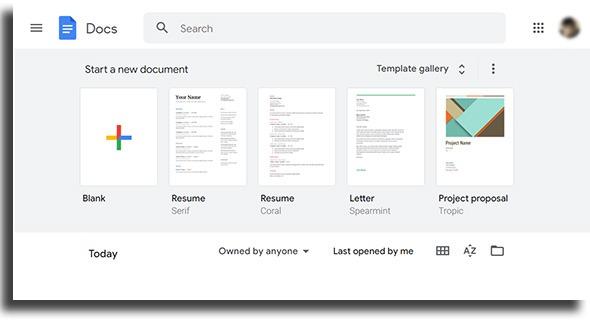**Website Interface Overview and Document Templates**

The interface features a sleek design with a dark black shadow encircling the website. Bands of black and white areas create a distinct visual contrast. Prominently, there is a dark blue piece of paper adorned with white lines and black text that reads "Docs."

Adjacent to this, a dark gray rectangle contains a black magnifying glass icon and dark gray text that reads "Search." Beyond this, there is a square composed of smaller, unjoined black squares.

Towards the center, a blurred silhouette of a user's profile picture is visible. Within a dark gray section, bold black text states "Start a new document." Below this, a multicolored cross within a white rectangle is split into four parts: red, orange, blue, and green, with the label "Blank" in bold black text beneath it.

Several templates are displayed:

1. **Resume Templates**:
   - The first resume template showcases the bold black text "Your Name" at the top, followed by placeholder text. It is labeled "Resume" in bold, and in gray text, it says "Serif."
   - The second resume template is simpler, also labeled "Resume" in bold black text, with "Corel" in gray below it.

2. **Cover Letter Template**:
   - This template features sections for an opening, body, and closing. The bold black text labels it as a "Letter" with "Spearmint" in dark gray below.

3. **Project Proposal Template**:
   - This template is designed with light blue, teal, tan, and orange blocks, accompanied by both bold and regular black text. It is labeled "Project Proposal" in bold black text, with "Tutorial" in gray underneath.

On the left-hand side, bold black text reads "Today," followed by regular black text "Owned by anyone" with a drop-down arrow, and "Last opened by me." There is also a black rectangle divided into six equal squares, featuring up and down arrows with "A to Z," likely for font adjustment or sorting. Adjacent to this is a black folder icon.